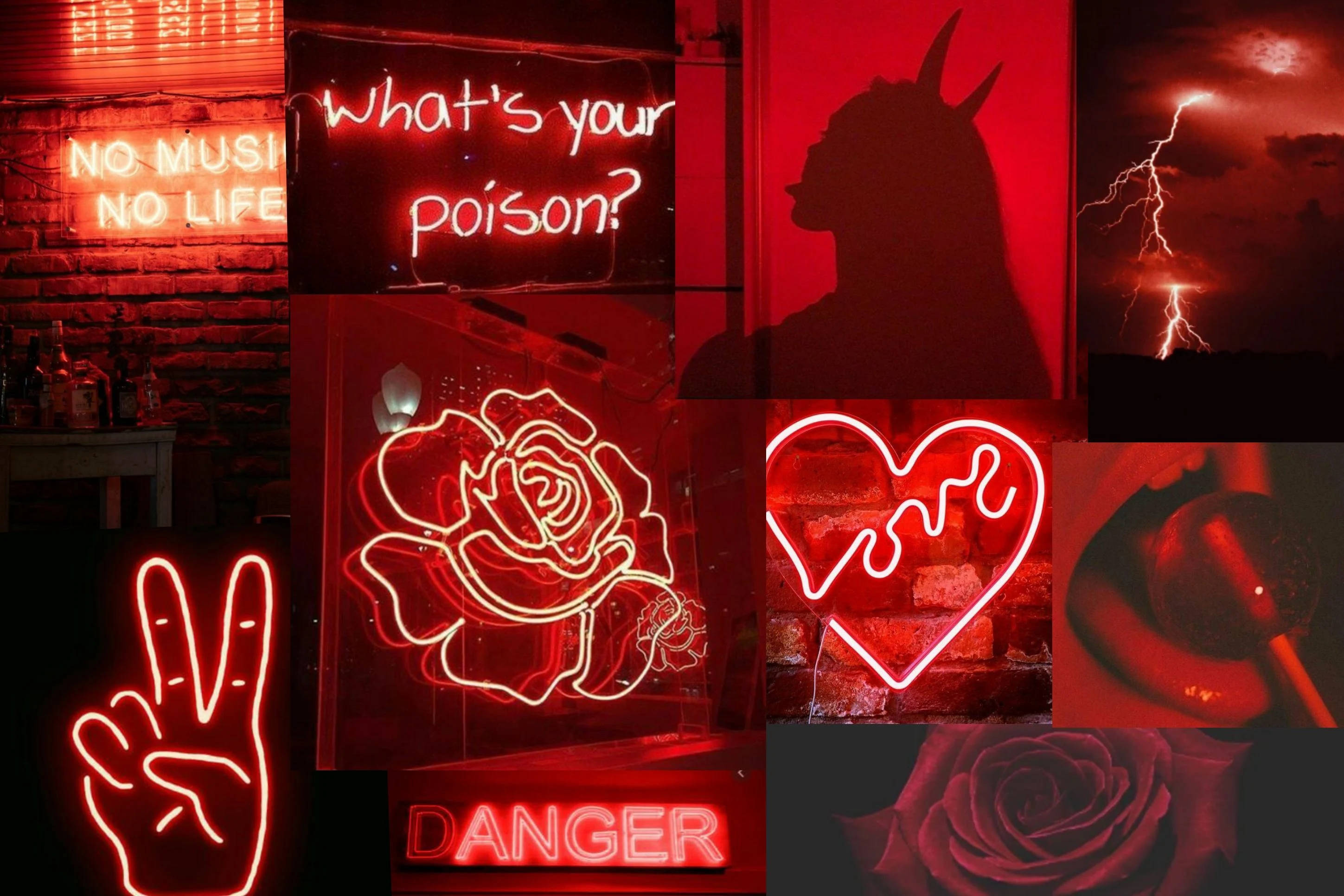A detailed collage of images, predominantly in shades of red and black, is featured, each with a distinct neon aesthetic. The upper left image showcases a neon sign reading “No Music, No Life” against a red brick wall, with various drinks arranged below. Adjacent to it, a bright neon sign asks, “What’s Your Poison?”, emphasizing a darker, mysterious allure. Below that, the silhouette of a devil-girl with horns and her tongue out casts a shadow against a vivid red wall. 

Close by, a spectacular red sky filled with a bolt of bright golden lightning contrasts against the dark backdrop. Further down, a radiant peace sign is displayed, followed by a striking neon rose with the word “Danger” inscribed beneath it, adding an element of caution. Additionally, a bold neon heart contains the word “Love”, illuminating the surroundings with a warm red glow. Completing the compilation is an evocative image showing a person, tinted in red light, savoring a lollipop, adding a playful yet sensual touch to the series.